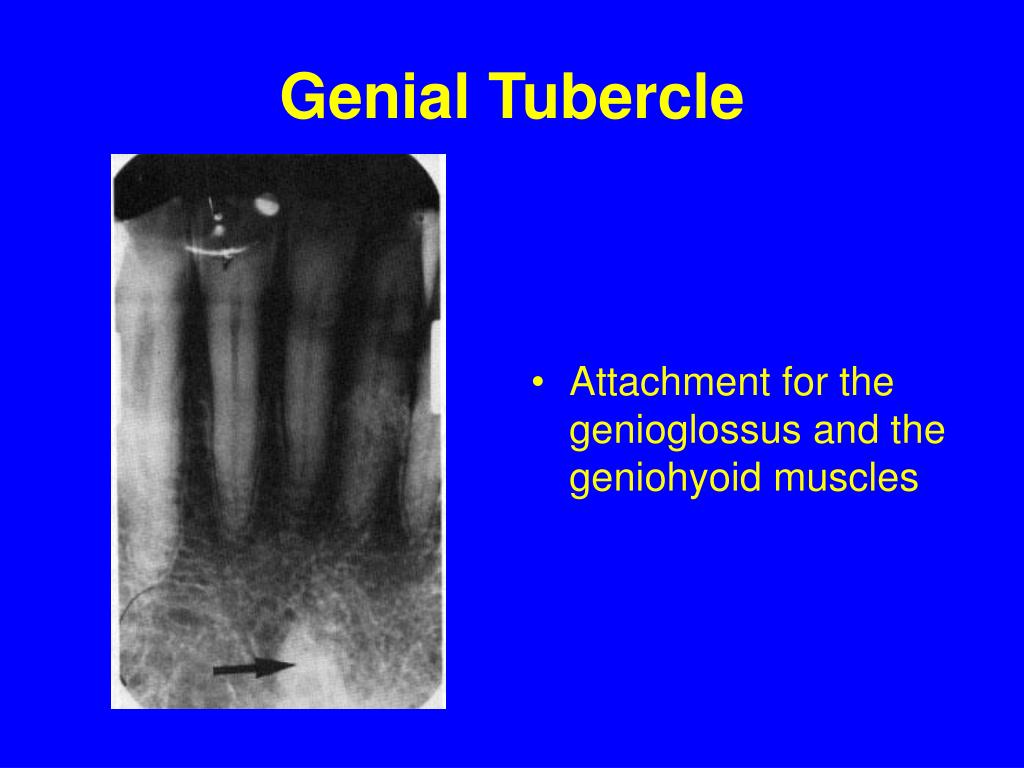This presentation slide features a detailed examination of the Genial Tubercle, highlighted in bold yellow letters at the top center against a solid bright blue background. The slide includes a black-and-white x-ray image positioned in the bottom left corner, showcasing a close-up view of a body part, likely dental in nature. This x-ray displays vertical white lines resembling teeth, with a small black arrow indicating a specific white spot identified as the Genial Tubercle. On the right side of the slide, there's a centered yellow bullet point that reads "Attachment for the Genoglossus and Genohyoid muscles," explaining the anatomical significance of the Genial Tubercle. The clear and structured layout with vibrant colors emphasizes the educational purpose of the slide, making it a useful tool for understanding this particular anatomical feature.